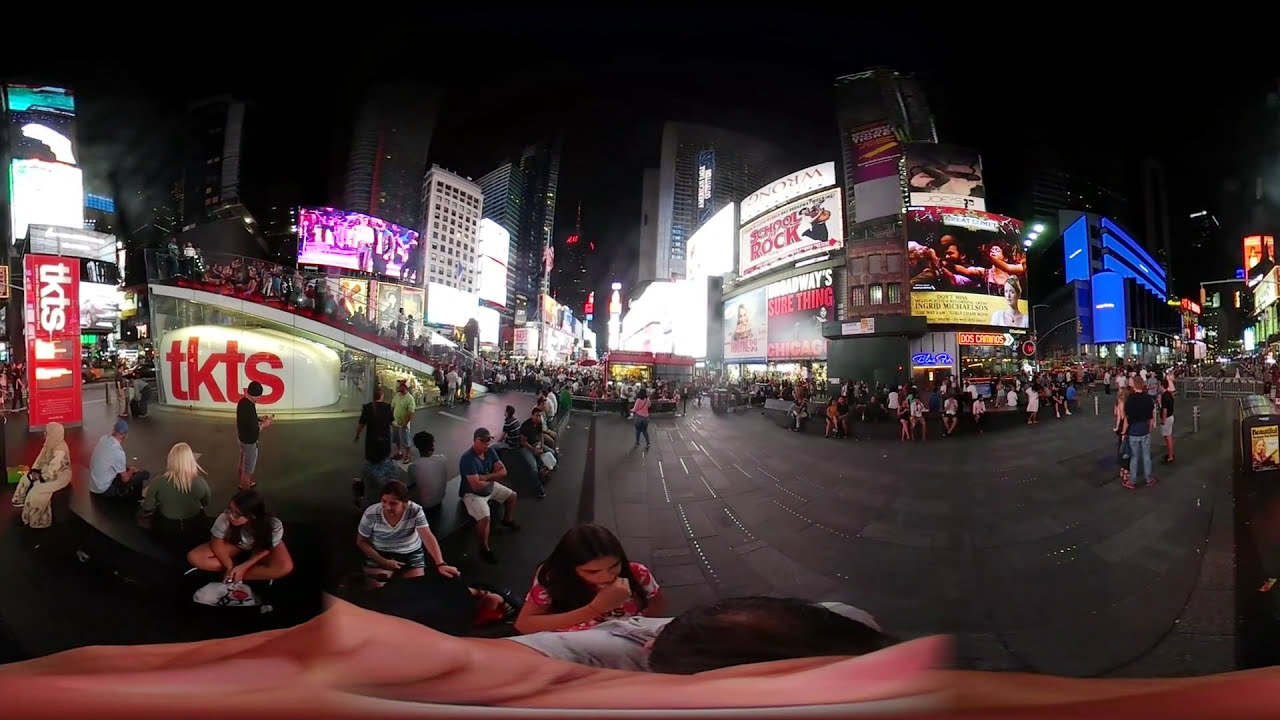The image captures a bustling theater district at night, illuminated by the vibrant and colorful lights from numerous buildings and advertisements. The ground is covered with concrete tiles, and various individuals are either sitting on benches or walking around. On the left side of the photo, people appear to be queuing up in front of a ticket booth, identified by the red letters "TKTS" on a white background. The center features a bright multicolored building adorned with billboards and screens, including a prominent "School of Rock" sign and another related to Broadway. The right side shows a vividly lit blue building. The crowd, composed of people with diverse hairstyles and attires in black, white, green, yellow, purple, pink, gray, tan, blue, and orange, is spread out across the scene, creating an energetic and festive atmosphere indicative of a major downtown area.